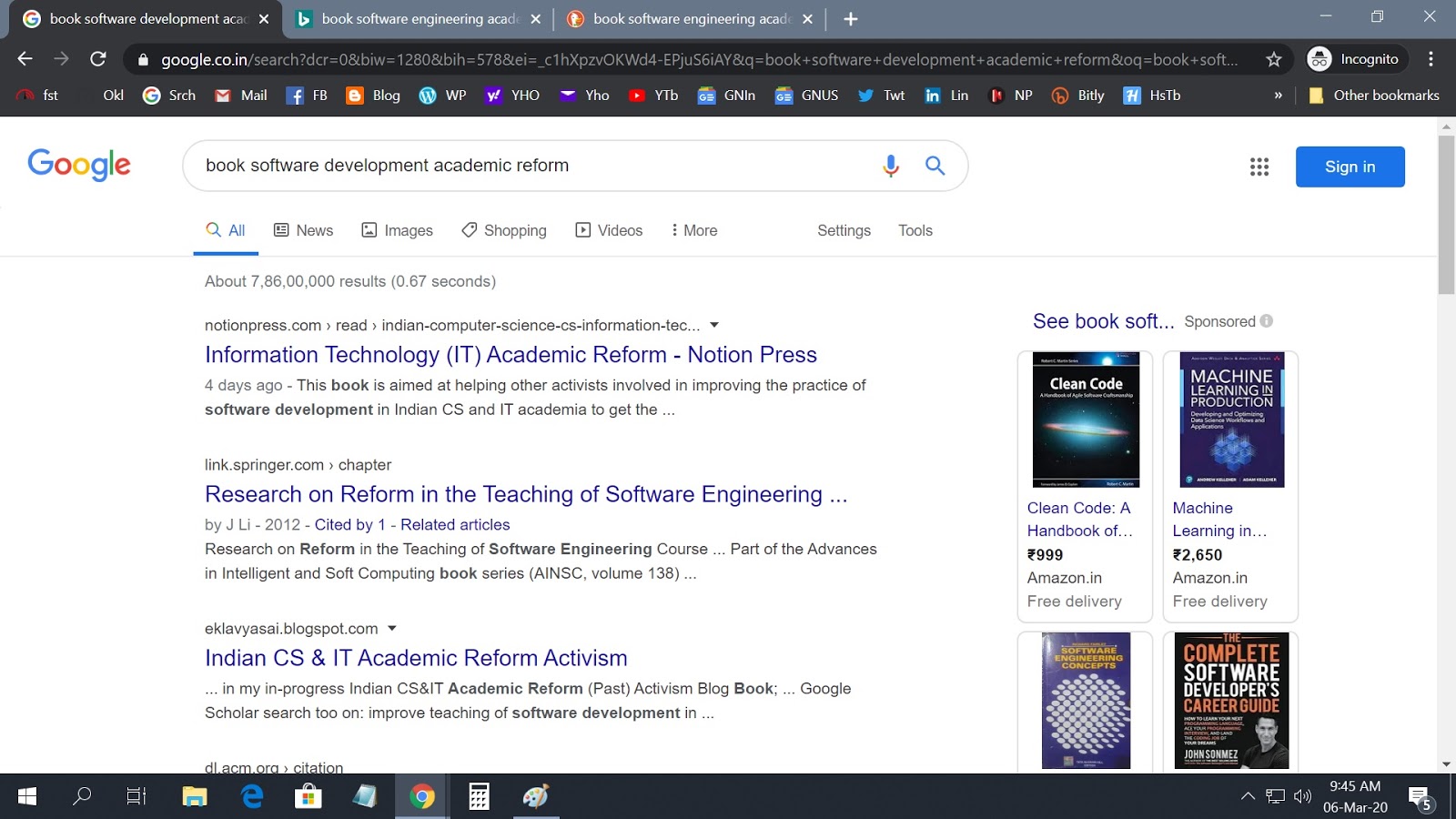This image depicts a screenshot of Google search results on a computer. The top portion features a bluish-gray header with two tabs on the center-left containing white text. The first tab is labeled "Book Software Engineering," while the rest of the text on both tabs is cut off. Nearby, on the top-left corner, there is a dark gray tab displaying the Google logo on the left and the cut-off white text "Book Software Development at Cat."

Below this header, there are several navigational elements: a white left-pointing arrow, a gray right-pointing arrow, and a white refresh button. To the right of these elements is a long URL bar with rounded ends, which holds a white lock icon on the left and a white star icon on the right. The URL bar is filled with text starting with "google.co.in/search?q=DCR=" followed by an extended URL string. Adjacent to the URL bar, on a dark gray button, the word "Incognito" appears in white text; next to it is a white circle containing a dark gray icon of a hat and glasses.

Beneath this header are numerous bookmarks, identifiable by their icons and white text labels. Below these bookmarks is the main body of the webpage, displayed against a white background. On the top-left part of this section is the colorful Google logo, and to its right is a white search bar filled with the black text "Book Software Development Academic Reform."

Further down, there are various tabs labeled "All," "News," "Images," "Shopping," "Videos," "More," followed by "Settings" and "Tools" after a bit of negative space. The "All" tab is highlighted in blue, adorned with a blue magnifying glass icon and an underlined blue text.

Finally, the screenshot includes the search results. To the right side of these results, book listings are presented, complete with prices, website links, and delivery cost information.